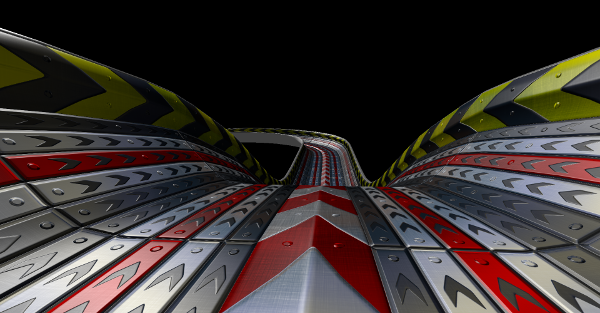The image depicts a CGI-rendered racetrack, reminiscent of those found in video games, set against a pitch-black background that suggests a floating structure with no visible sky. The track comprises two lanes separated by a prominent, raised center divider adorned with a red and white chevron pattern. The surface of the track alternates between gray, silver, and red, and is intermittently segmented with varying chevron motifs. Along the outer edges of the track, tightly packed guardrails featuring black and yellow warning chevrons are present. 

Forward-pointing arrows are visible in different areas, with a mixture of silver, gray, and yellow arrows populating the track, emphasizing the direction of movement. The track itself appears to extend into the distance, curving sharply to the left, suggesting a dynamic and challenging course. The vivid color palette, including shades of black, red, white, silver, and yellow, contributes to the overall industrial, high-tech aesthetic of this fantastical racing environment.